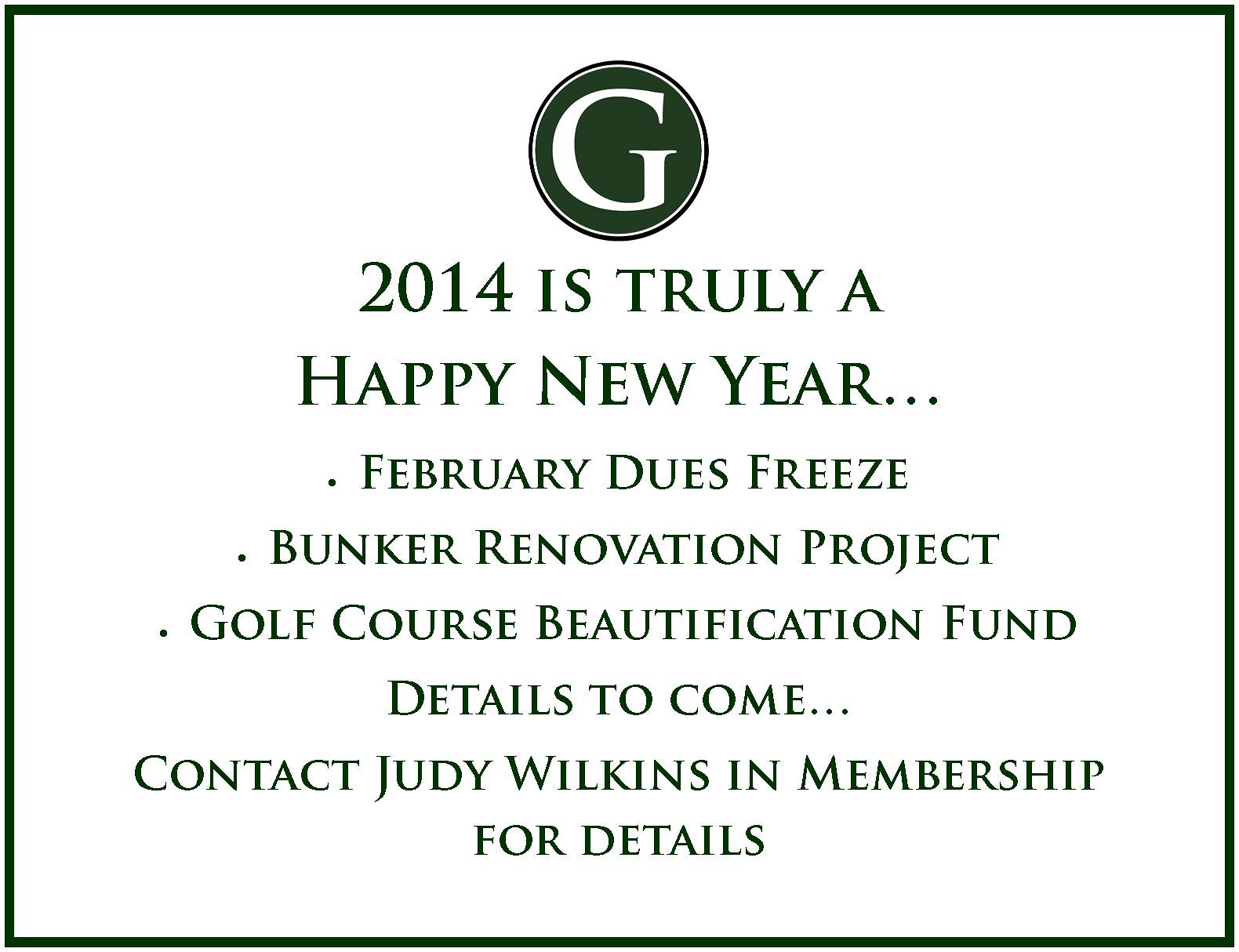This image is a computer-made graphic with a predominantly white background bordered by a thin, dark-colored border. At the very top of the image, there is a circular logo featuring a large white letter "G" inside. The background of the circle matches the color of the border, either black or dark blue. 

Below the logo, the text "2014 is truly A Happy New Year" is center-aligned, written in capital letters. This is followed by a bullet-pointed list, also center-aligned and in the same color as the border. The list includes the following announcements:
- February dues freeze
- Bunker renovation project
- Golf course beautification fund (details to come)

At the very bottom of the image, without a bullet point, it reads: "Contact Judy Wilkins in membership for details." The entire layout is clean and structured, providing essential information concisely and clearly.